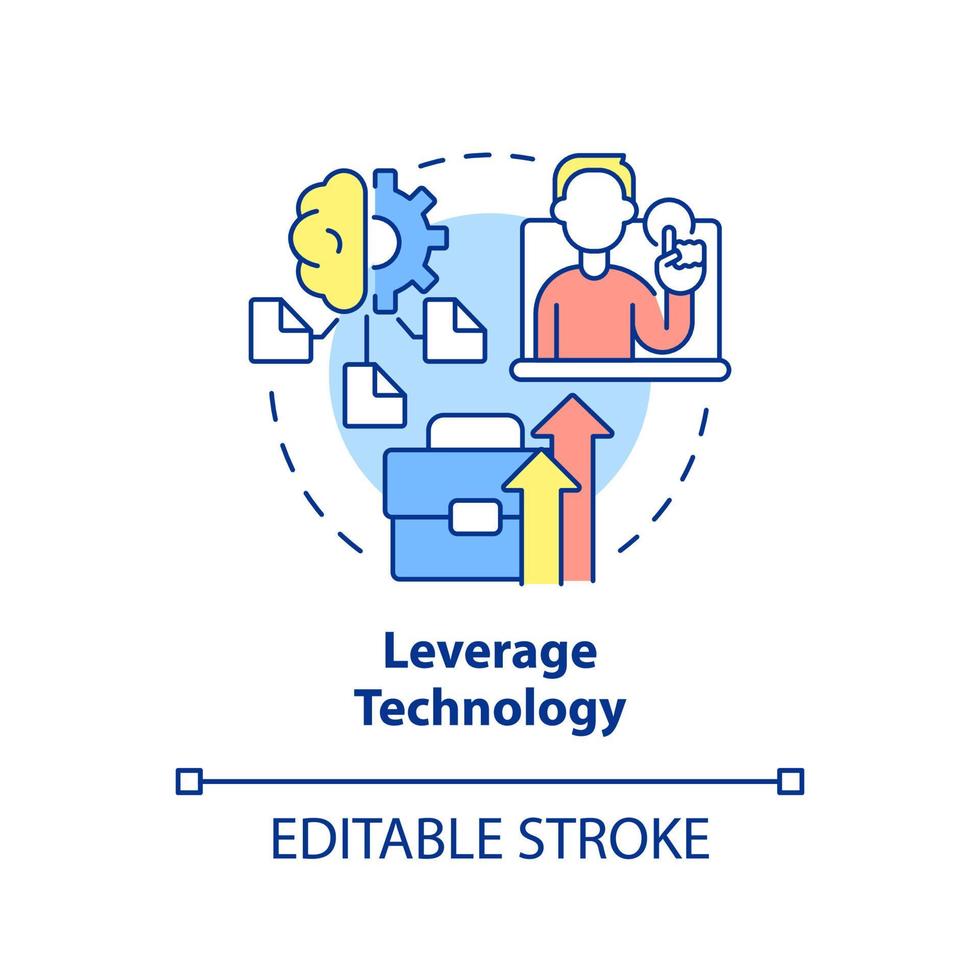This is a detailed digital illustration consisting of various interconnected elements, all set against a white background. At the center of the illustration is a large light blue circle enclosed within a dotted circle. Overlaid on this is a gear that appears to be connected to three smaller pages, each with a dog-eared corner.

To the top right within the dotted circle is an illustration of a person with yellow hair, wearing an orange sweater, and raising their left hand with the index finger pointing upwards. This figure has no facial features. 

Below this central configuration is a light blue briefcase symbol, positioned at the bottom of the dotted circle. Two arrows are seen pointing upwards from the briefcase—one yellow and one pink.

At the very bottom of the illustration, the words "Editable Stroke" are written below a horizontal blue line, which extends from left to right with small blue boxes at each end. Above this line, centered in blue text, is the phrase "Leverage Technology."

The entire composition is rendered in shades of blue, yellow, and pink, and seems to represent a thematic diagram, possibly conveying concepts related to technology and its applications.